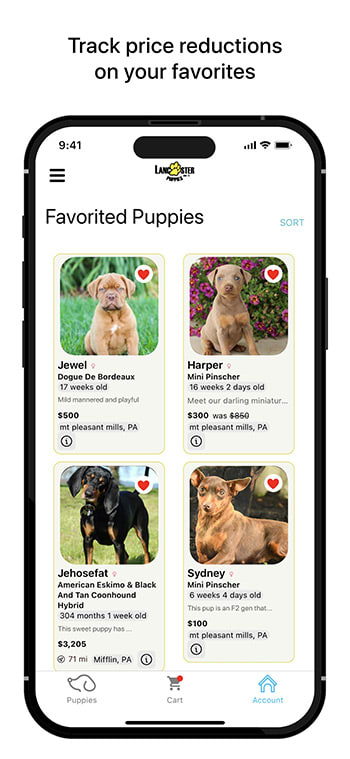The image showcases an iPhone against a clean, white background. The phone screen displays the Lancaster Puppies app. At the top-left corner of the screen, the time reads 9:41. The top-right corner indicates full service, full Wi-Fi, and a fully charged battery. The app's title, "Lancaster Puppies," is centrally positioned with a yellow paw print between the words "Lancaster" and "Puppies," both in black font. The menu is represented by three horizontal bars towards the top left.

Below the app title, there's a black text label "Favorited Puppies" and a blue "Sort" option to its right. The screen showcases a grid layout of four puppies, arranged in two rows and two columns: Jewel, Harper, Jehoshaphat, and Sydney.

Detailed descriptions of each puppy are visible:
- **Jewel**: A Dogue de Bordeaux, 17 weeks old, described as mild-mannered and playful, priced at $500, located in Mount Pleasant Mills, PA.
- **Harper**: A Miniature Pinscher, 16 weeks and 2 days old, labeled as "Meet Our Darling Miniature," with a reduced price of $300 from $850, also located in Mount Pleasant Mills, PA.
- **Jehoshaphat**: An American Eskimo and Black and Tan Coonhound Hybrid, 304 months and 1 week old. The description is partially cut off but notes this "sweet puppy," priced at $3,205, located 71 miles away in Mifflin, PA.
- **Sydney**: Another Miniature Pinscher, 6 weeks and 4 days old, described as an F2 Generation pup, priced at $100, in Mount Pleasant Mills, PA.

Each puppy listing includes an informational "i" icon at the bottom-left corner. At the bottom of the app, a menu features options for "Puppies," "Cart," and "Account," with "Account" highlighted in light blue to indicate the current selection.